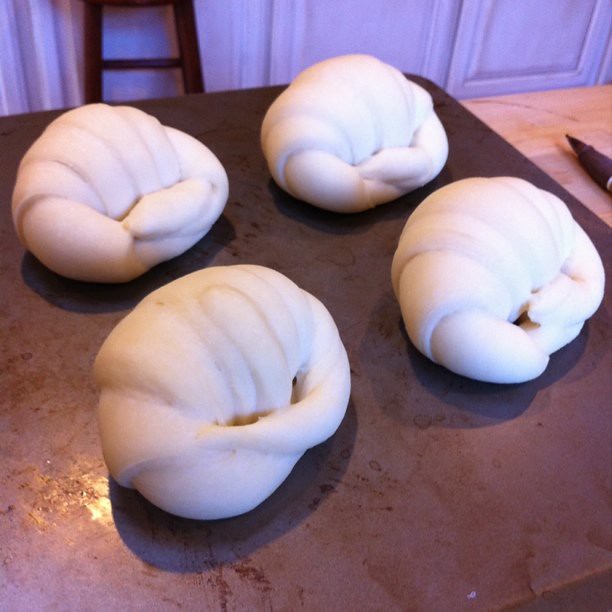The image depicts four large, uncooked croissants made from white dough, each shaped like a classic croissant. These raw pastries are placed on a dark brown cookie sheet, which is positioned on a light wooden countertop. In the background, white cabinets and the legs of a brown stool are visible, adding to the kitchen setting. The dough, light tan in color, appears smooth and ready for baking.